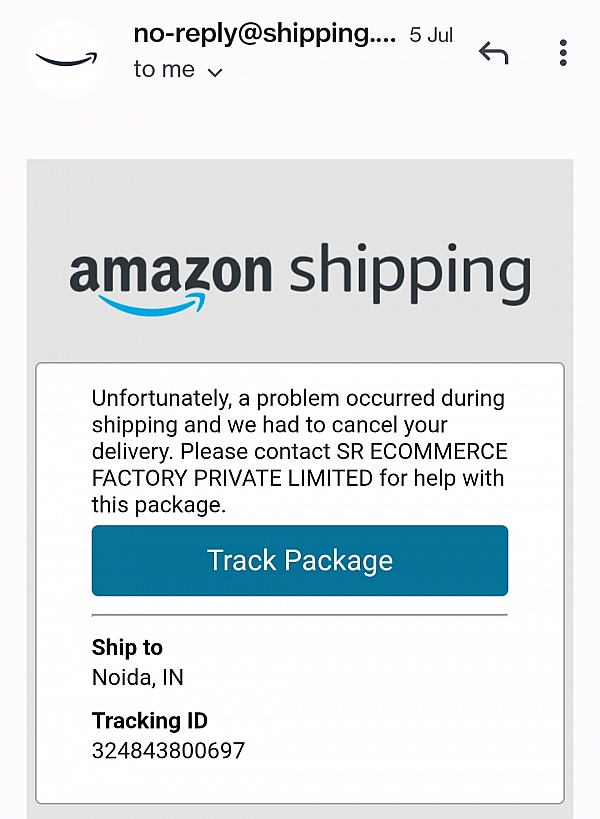The image is a screenshot taken on a mobile phone. The background at the top and along the left and right sides is a very pale gray. At the top of the screen, it reads "no reply," displayed next to the Amazon arrow icon. Below this, there is text that says "to me," and at the upper right corner, there are an arrow icon and a three-dot menu icon.

The central part of the image features a slightly darker gray box. At the top of this box, in large font, it says "Amazon shipping" with a blue arrow underneath. Below this, there is a white pop-up box that states, "Unfortunately, a problem occurred during shipping and we had to cancel your delivery. Please contact SRE Commerce Factory Private Limited for help with this package." 

At the bottom of this white box, there is a long, horizontal dark navy blue button with the text "Track package" in white font. Below the button is a thin gray horizontal line. In the lower left corner, bold text reads "Ship to" and "Tracking ID." The "Ship to" section indicates Noida, Indiana, and the "Tracking ID" is 324843800697.